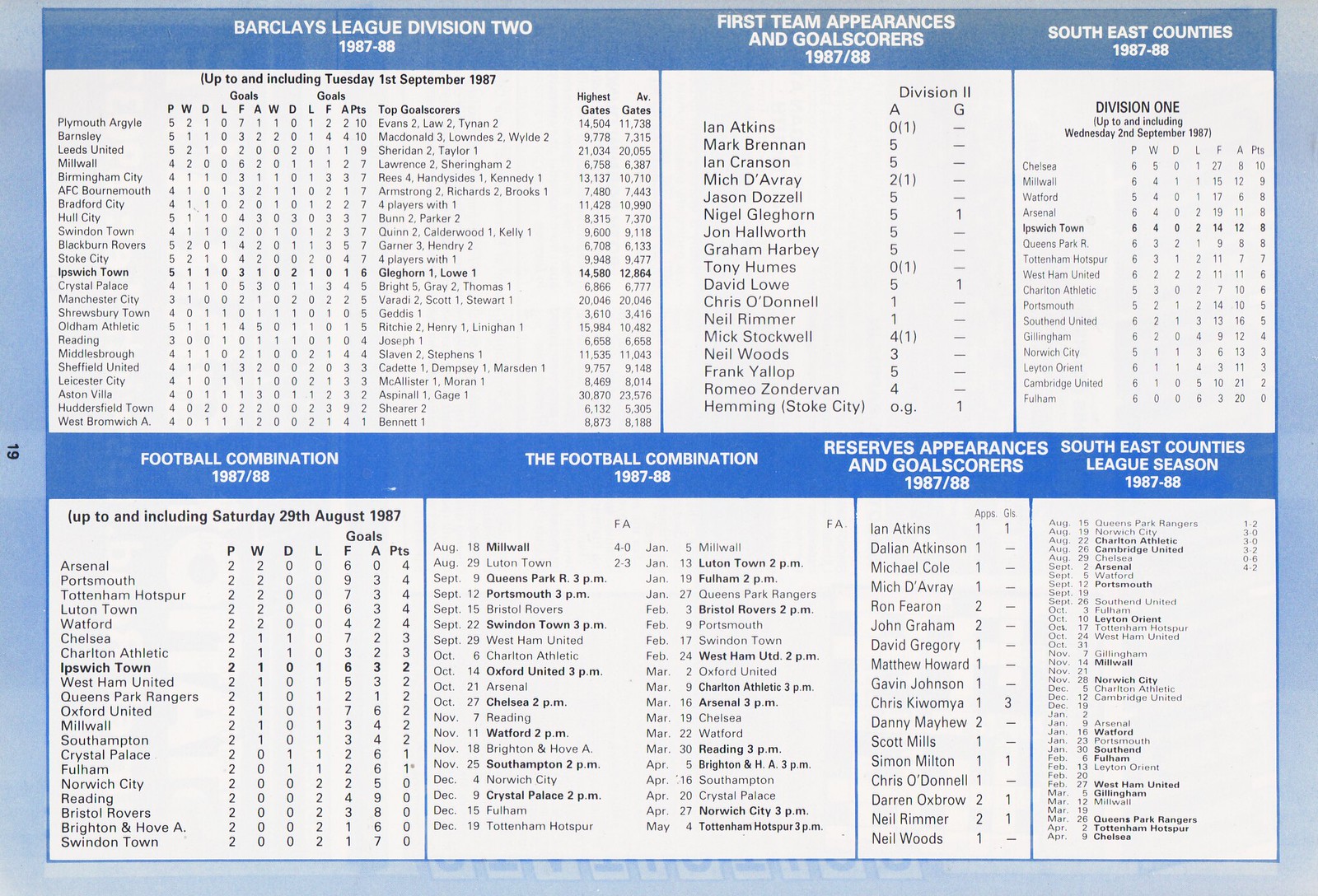This image is a horizontal page from a game day program, specifically page 19, which meticulously charts various football scores and statistics for the 1987-88 season. It features several detailed tables, each separated by blue borders and accentuated by headings in blue bars against a light sky blue background. The sections include "Barclays League Division II 1987-88," "First Team Appearances and Goal Scores 1987-88," "Southeast Counties 1987-88," "Football Combination 1987-88," "Reserves Appearances and Goal Scores 1987-88," and "Southeast Counties League Season 1987-88." Each table documents teams' wins, losses, scores, and additional performance metrics. Notably, "Ice Pitch Town" appears in a darker font, suggesting it is the primary focus of the chart. A barely readable watermark is located at the bottom of the page.